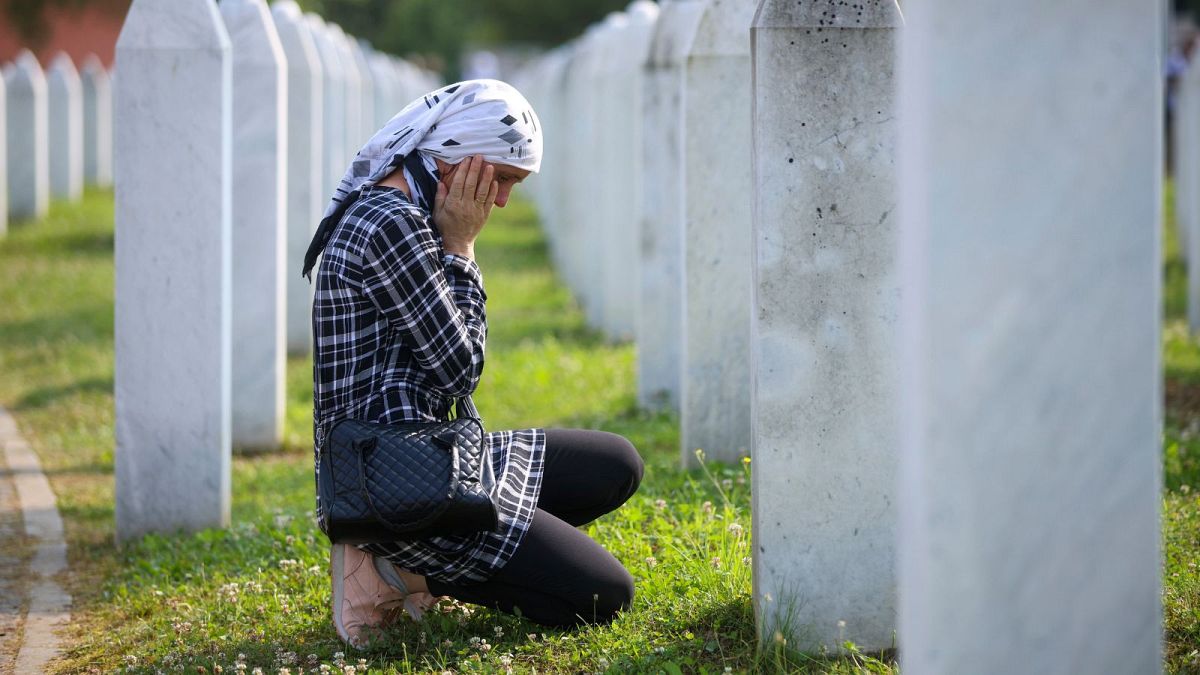The image depicts a solemn, outdoor setting of a large military cemetery characterized by rows upon rows of identical, white, thin, tall, and pointed headstones. These headstones, likely made of light gray stone, form a repetitive, uniform pattern, emphasizing the vast number of fallen soldiers honored there. In the foreground, a woman is kneeling on the neatly kept grass, deeply immersed in mourning. She has her hands pressed against her cheeks, conveying an overwhelming sense of grief and loss, as if she might be crying. Dressed in a long-sleeve, navy plaid tunic shirt that extends to her thighs, black leggings, and pink tennis shoes, her attire is modest and somber. A white scarf with blue and gray designs covers her head. A black handbag hangs from her shoulder, resting against her side. The scene captures the profound and personal sorrow amidst the collected memories of countless soldiers, in a space designed for quiet reflection and remembrance.